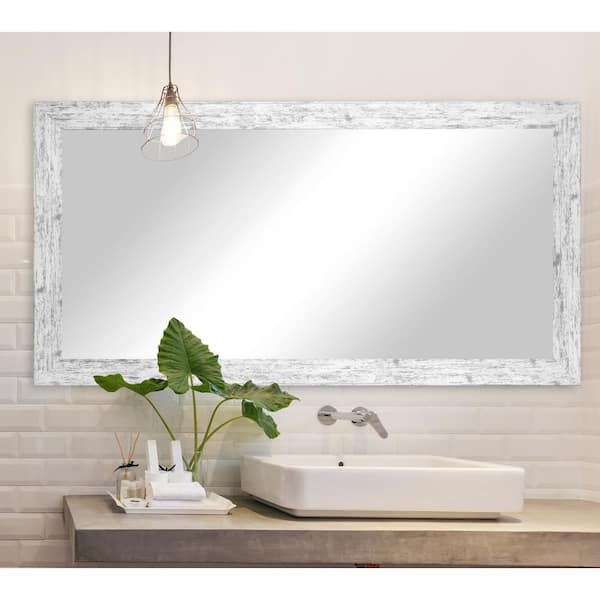The image captures a serene bathroom with a blend of modern and rustic elements, featuring a prominent white brick tiled wall. Central to the scene is an elegantly large mirror framed in ashy white wood, which reflects the room’s light, giving it a spacious feel. Hanging above the mirror, an old-fashioned, exposed light bulb encased in a protective cage illuminates the area. Below, the focal point is a striking, square white basin sink, perched on a light brown faux wood countertop. The water fixture extends directly from the tiled wall into the sink. To the left of the sink, a small yet vibrant plant, resembling elephant ears, injects a lively burst of green into the predominantly neutral palette of beige, white, and gray tones. Complementing the plant is a dish holding various items, including a possible bar of soap and personal effects, as well as a set of rolled-up towels and fragrance reed diffusers, offering a subtle touch of sophistication akin to a high-end hotel. The overall scene is clean, minimalistic, and tastefully detailed, creating a restful and stylish bathroom atmosphere.